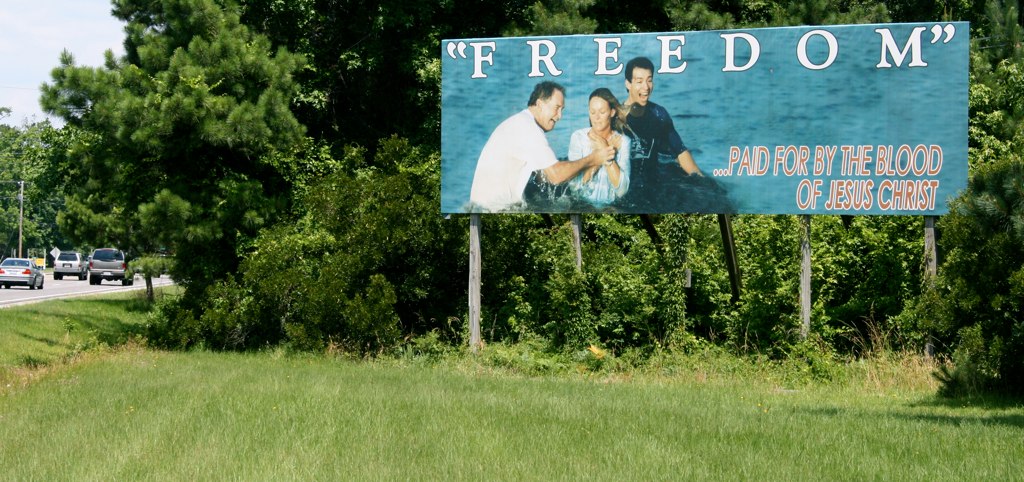In the image, lush green grass covers the foreground, with a collection of trees and bushes lining the right side. To the left, three vehicles are visible on the adjacent street: a car and two SUVs. Dominating the left portion of the scene is a large billboard. The billboard bears the word "Freedom" and features an image of a girl being baptized. She is dressed in light blue, with a man in dark blue standing behind her and presumably a preacher, dressed entirely in white, standing in front of her, guiding the baptism. Below the image, the text "Paid for by the blood of Jesus Christ" is displayed in red, punctuated by ellipses. The billboard is supported by four rectangular, pyramid-shaped poles. In the background, a few power lines stretch across the horizon, enhancing the depth of the scene.